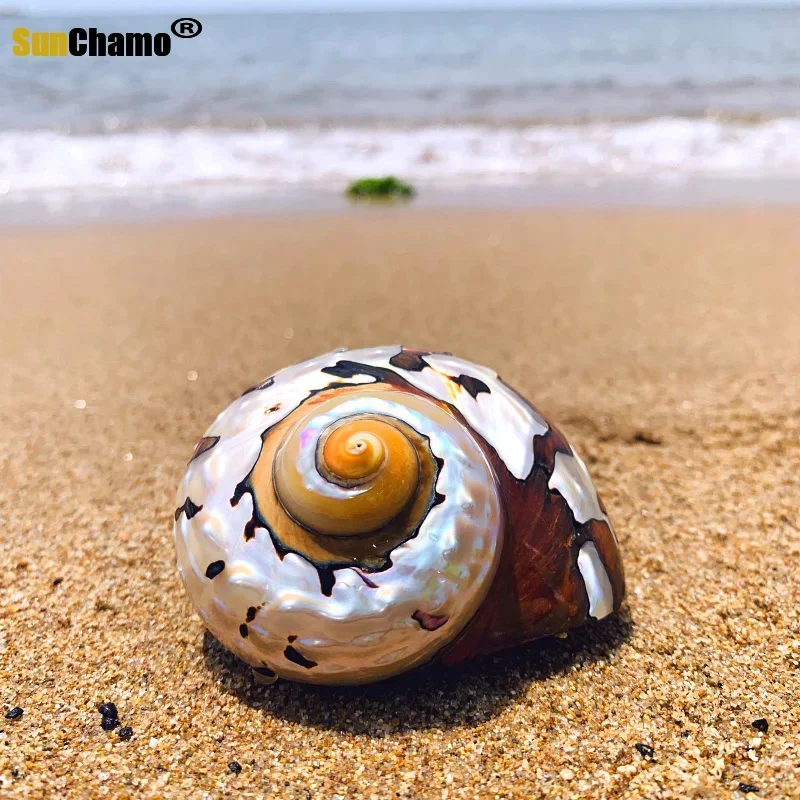This photograph captures a mesmerizing beach scene under the midday sun. The image, square in shape, prominently features a luminescent, pearlescent shell in the clear, detailed foreground. The shell, resembling a nautilus, spirals inward with a pearly finish accented by brown speckling and a caramel hue at its rounded center. Its intricate design casts a defined shadow forward, highlighting the light source from behind. The sand beneath the shell is a tan, dusty color interspersed with black sand particles.

As the focus shifts backward, the scene becomes beautifully blurred, showcasing an indistinguishable green object amidst the soft waves of the ocean. High above, the sun is at its zenith, casting a serene and bright atmosphere over the setting. The upper left corner of the image bears the bold text "Sun Camo" in a sand-surf typeface, with "Sun" rendered in yellow and "Camo" in black, accompanied by a registered trademark symbol in the top right corner. This immersive beach snapshot perfectly blends the tranquility of the ocean with the delicate detail of the shell.